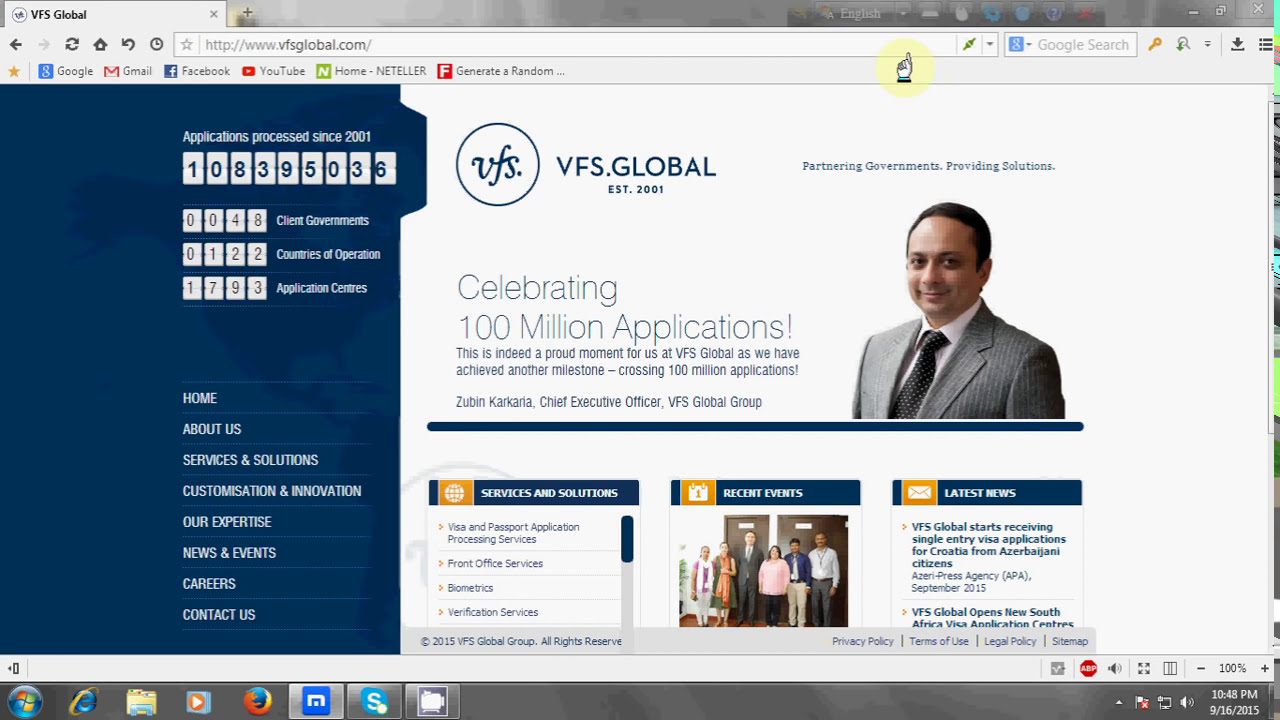This image is a detailed screenshot of a VFS Global web page. The web browser tab is labeled "VFS Global". Below the tab, the navigation bar contains a back arrow, an inactive forward arrow, a refresh button, a home button, a return button, and a clock icon. The URL displayed in the search bar is "http://www.vfsglobal.com," accompanied by a lock icon indicating a secure connection.

In the center of the screen, a yellow circle highlights a hand icon with an index finger pointing at the search bar. The webpage's main content is divided into thirds horizontally. The left third features a dark blue section with white text, stating various statistics:

- Applications processed since 2001: 108,395,036
- Client governments: 48
- Countries of operation: 122
- Application centers: 1,793

Each statistic is presented in individual white boxes with dark text. Below these statistics, navigation links are listed in white text: Home, About Us, Service and Solutions, Customization and Innovation, Our Expertise, News and Events, Careers, and Contact Us.

The right two-thirds of the page feature the VFS Global logo, a blue circle with "VFS Global" in blue uppercase letters and the tagline "Established 2001, Partnering Governments, Providing Solutions." Below the logo is a photograph of a clean-shaven man with dark hair wearing a gray pinstripe suit, white shirt, and tie. The accompanying text celebrates the milestone of processing over 100 million applications, with a message from Zubin Karkaria, Chief Executive Officer, VFS Global, written in blue.

A dark blue bar spans the width of the screen below this section, followed by three informational boxes:

1. The first box has an orange icon of a globe and is titled "Services and Solutions" in blue letters on white. It lists services including Visa and Passport Application Processing Services, Front Office Services, and Biometrics and Verification Services, each with a right-facing orange arrow.
2. The second box, with an orange calendar icon, is titled "Recent Events" in white uppercase letters. It features an image of six people standing in front of doors.
3. The third box has an orange envelope icon and is titled "Latest News." It includes two news items:
   - VFS Global starts receiving single entry visa applications for Croatia from Abidjani citizens (Abidjan Press Agency, September 2015).
   - VFS Global opens New South Africa Visa Application Center.

At the bottom left, the page displays "Copyright 2015, VFS Global Group, All Rights Reserved." On the bottom right are links to the Privacy Policy, Terms of Use, Legal Policy, Sitemap, and other standard footer elements.